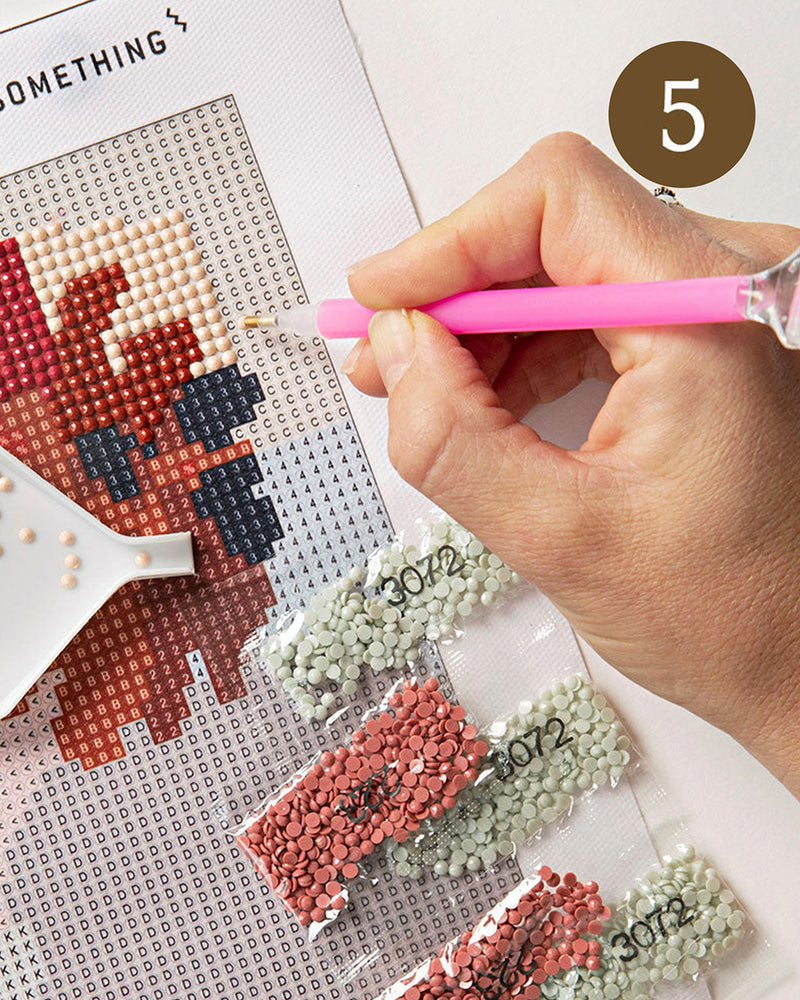In this detailed photograph, a person with light, pale skin, presumably Caucasian, uses a pink pen to meticulously place tiny, colorful pellet beads onto a mat that features small dents, creating a pixel-like piece of artwork. At the top of the mat, in bold capital letters, it reads "JOURNEY OF SOMETHING." The hand, firmly grasping the pink pen, seems to be arranging lighter pink or beige beads, while various other colored pellets, including black, green, red, and white, are already integrated into the design. These arranged beads potentially depict flowers or characters with distinct features. The completed design is intended to be fused together using an iron to form a cohesive image. Additionally, in the upper right corner of the image, a number "5" is displayed within a brown circle. Below the mat are bags containing assorted color pellets, ranging from white to pink, ready for use in the artwork.